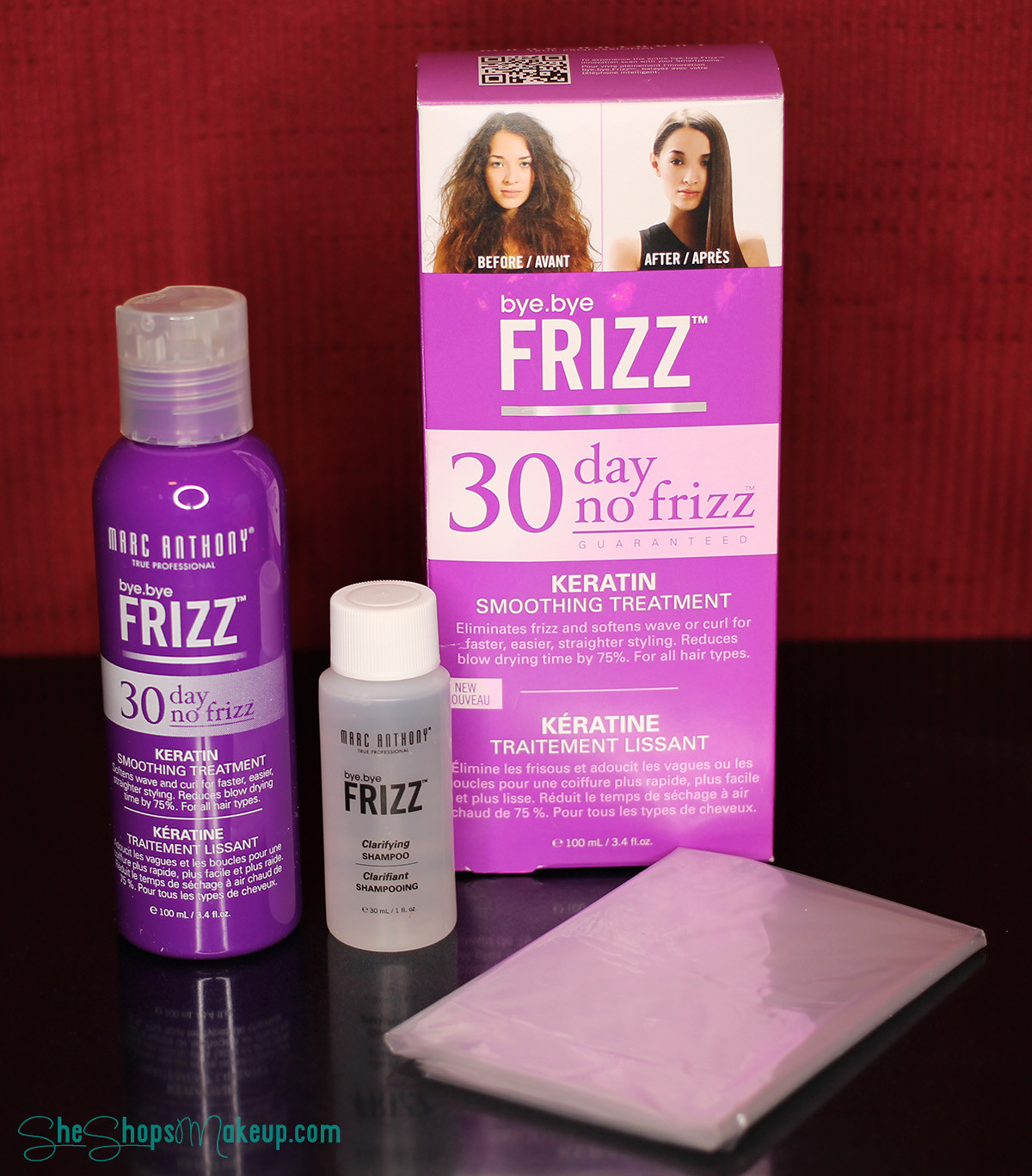This image showcases a comprehensive haircare kit against a vibrant red background, containing three key products aimed at taming frizz. Central to the display is a tall purple and white box labeled "Bye Bye Frizz" and "30 Day No Frizz Keratin Smoothing Treatment." The box features a striking transformation photo, depicting a woman with frizzy brown hair in the "before" picture and sleek, straight hair in the "after" image. The packaging proudly claims to eliminate frizz, soften waves or curls, and reduce blow-drying time by 75% for all hair types. 

Alongside the box are two bottles from the kit: a small transparent bottle with a white cap labeled "Frizz Clarifying Shampoo," and a larger purple bottle with a white top, also branded "Bye Bye Frizz 30 Day No Frizz Treatment." Additionally, the package includes a packet presumed to contain white tissue or additional items, enhancing the kit's comprehensive nature. The product collection is marketed by Marc Anthony, with a website for purchase information prominently displayed in the lower left-hand corner, reading "TheShopsMakeup.com."